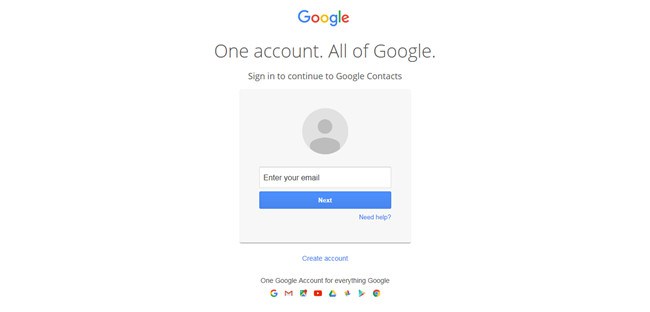This image is a screenshot of a Google sign-in page designed for mobile, though it lacks any specific mobile device UI elements. The interface features a clean, white background and a vertical layout typical of mobile screens. 

At the top center, the iconic Google logo is displayed, featuring the blue G, red O, yellow O, blue G, green L, and red E. Below this logo, there is a space followed by a centered heading in large, sans-serif, dark gray letters: "One account. All of Google." 

Further down, there's a subheading in smaller paragraph text that reads, "Sign in to continue to Google Contacts." Immediately beneath this, a light gray box houses a gray circle with a dark gray icon of a person, representing an avatar placeholder. 

Below the avatar, there's a field for entering an email address, which is white with a gray border and aligned center. Directly under this field is a blue rectangular button with the word "Next" in white letters, also centered and matching the width of the email field above.

On the right side below the button, a "Need help?" link is present. Underneath this, a thin horizontal line, approximately two or three pixels wide, divides the screen. 

Continuing down, the white background persists. In the center, a blue link reads "Create account." A small gap separates this from the subsequent small text that says, "One Google Account for everything Google." 

At the bottom, there are icons representing various Google applications: Google Account, Gmail, an unrecognized icon, YouTube, Drive, another unrecognized icon, Play Store, and Chrome.